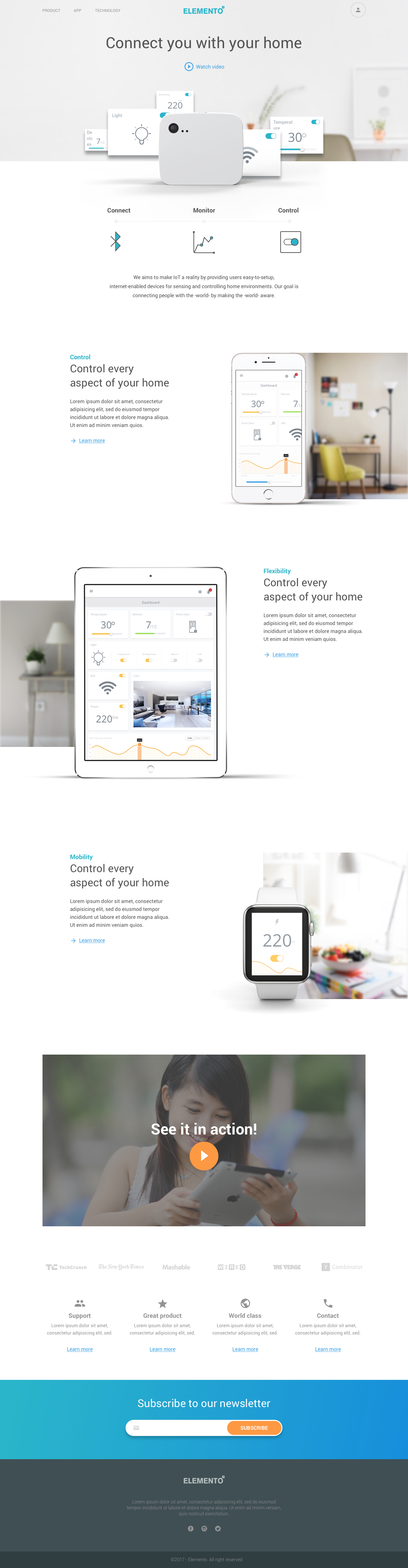This screenshot showcases a comprehensive home networking system designed to integrate seamlessly with your home environment. It features capabilities for managing temperature, WiFi, and lighting, offering users an easy setup for internet-enabled devices that monitor and control various household elements. The system aims to connect people more closely with their surroundings by providing accessible and intuitive tools for smart home management. The interface prominently encourages users to "Control Every Aspect of Your Home," emphasizing flexibility, mobility, and world-class support. Additional elements include options to see the product in action, contact support, and subscribe to a newsletter, inviting users to input their email and stay updated on new features and updates.